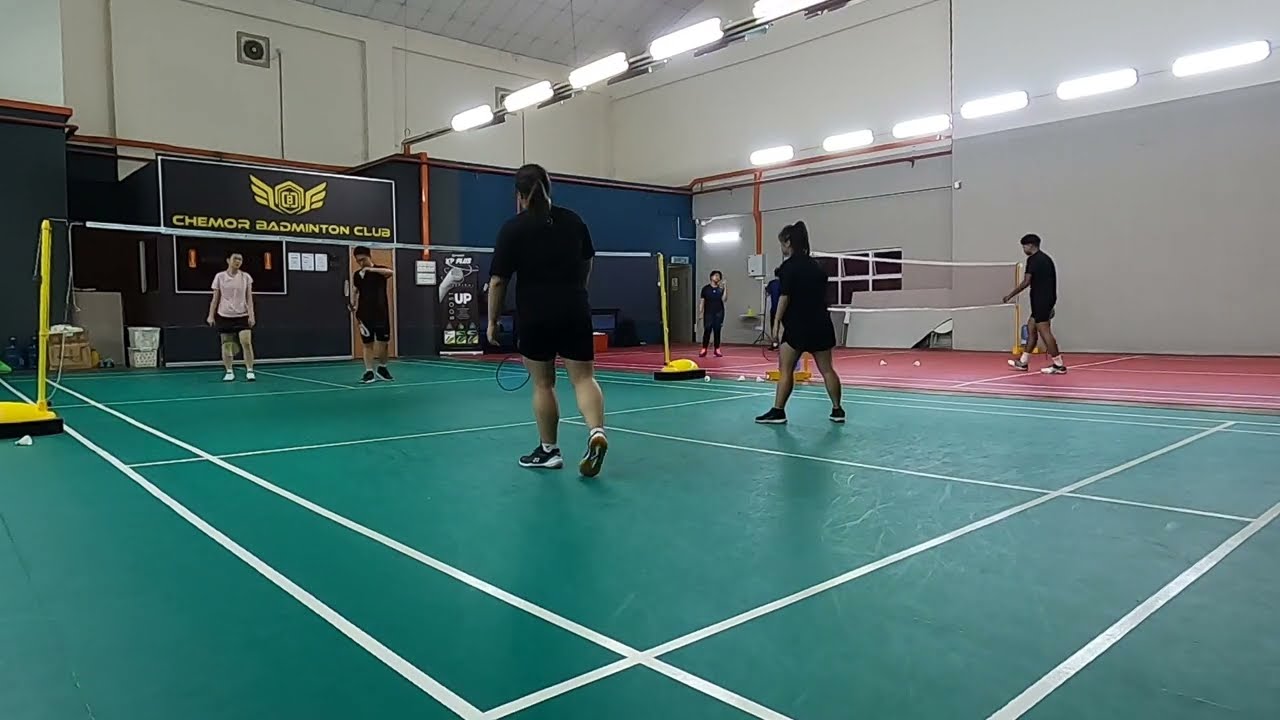The image depicts an indoor badminton game taking place at the Chemor Badminton Club, as indicated by a sign that reads "CHEMOR BADMINTON CLUB" in black with a yellow logo. The facility features multiple courts, including a green court with white lines and a red court. Both courts are equipped with a white and black net supported by yellow poles. The players, who appear to be of Asian descent, are engaged in matches with two on two on the green court and two players on the red court. The women in the foreground wear black shorts and black t-shirts, while on the opposing side, a man in black attire pairs with a woman in a pinkish top. The indoor auditorium is brightly lit from above and has white walls, contributing to a well-lit environment for the games.